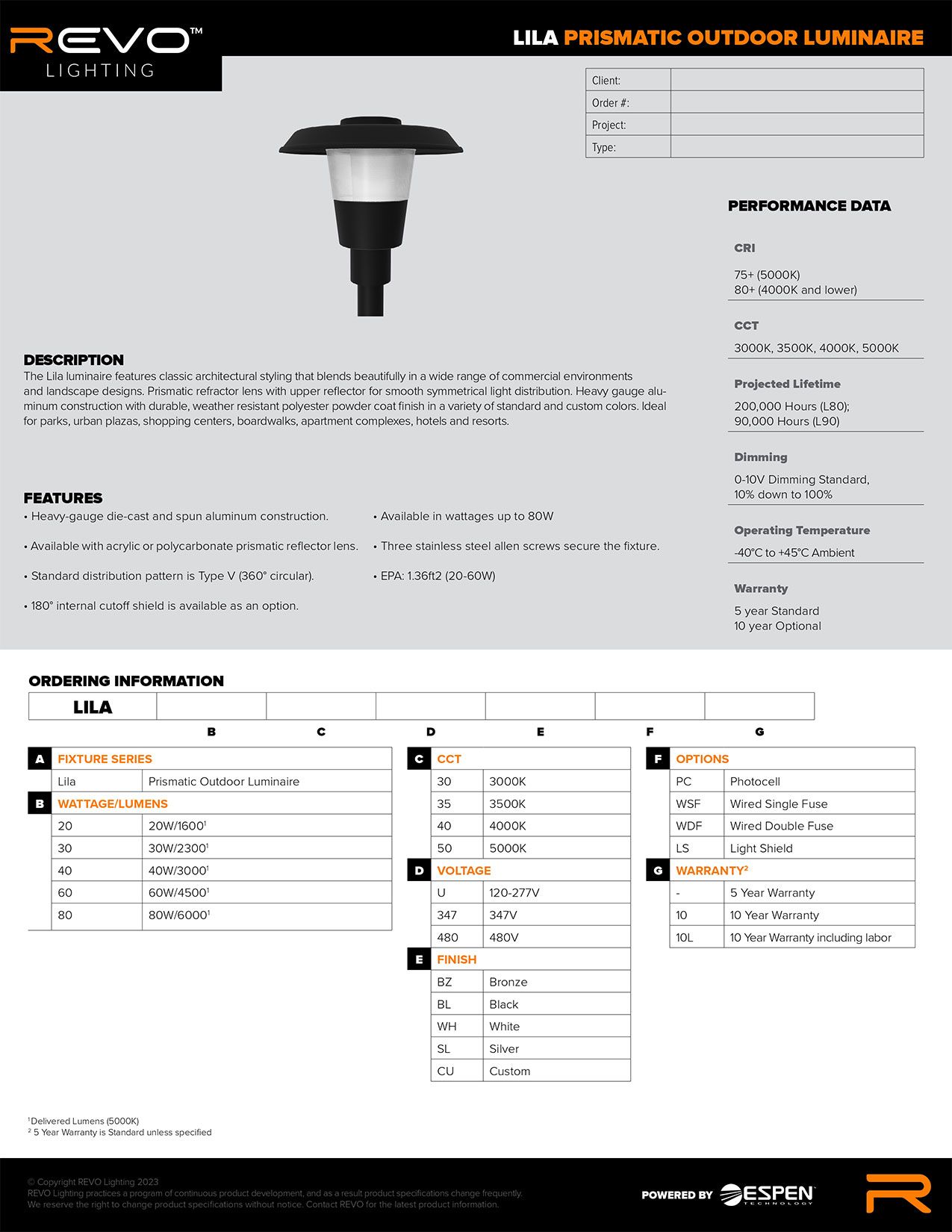The image displays a product page for Revel Lighting's Leela Prismatic Outdoor Luminaire. In the upper left-hand corner, the Revel Lighting logo is prominently featured, with a stylized "R" in orange and the remaining letters in white. The product name "Leela Prismatic Outdoor Luminaire" is shown beneath the logo, with "Leela" in white text and "Prismatic Outdoor Luminaire" in orange text.

In the top right corner, there is a table with columns labeled "Class" and "Type," although the values are not filled in. Below the table, there is an area designated for performance data. The middle section of the page contains a detailed paragraph description of the product. Lastly, beneath the description are seven bullet points, each highlighting a distinct feature of the Leela Prismatic Outdoor Luminaire.